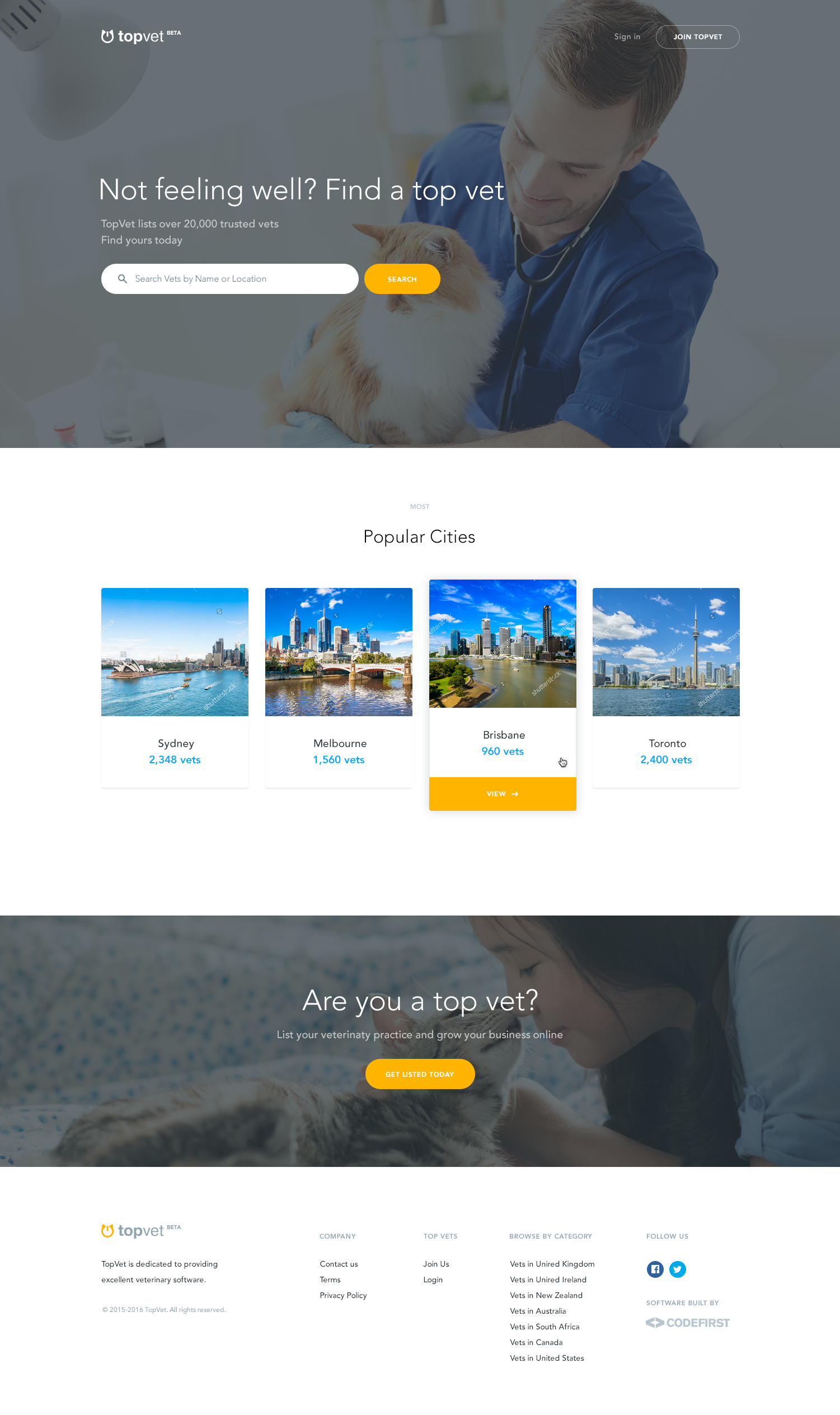The image features a gray box at the top, casting a shadow over the scene. Below it, a photograph captures a young veterinarian in blue scrubs, with brown hair and a stethoscope around his neck, attentively examining a long-haired cat. The cat's fur is predominantly reddish with a white chest, though its face is obscured by an orange bar. To the left of this bar, there's a white search bar.

Centered on the image, text reads, "Brought to you by Top Vet," followed by the tagline, "Not feeling well? Find a Top Vet." There's additional text that is too small to be legible. Underneath, the caption lists "Popular Cities," with accompanying pictures of four cities. The first two cities are Sydney and Melbourne, but the names of the third and fourth cities are unreadable. Below the third city, there's an orange box, likely clickable, indicating user interaction. 

Towards the bottom, another message asks, "Are you a Top Vet?" beside an orange bar that invites further engagement. The footer includes options to "Join us" or "Log in," along with additional information and social media buttons for Twitter and Facebook.